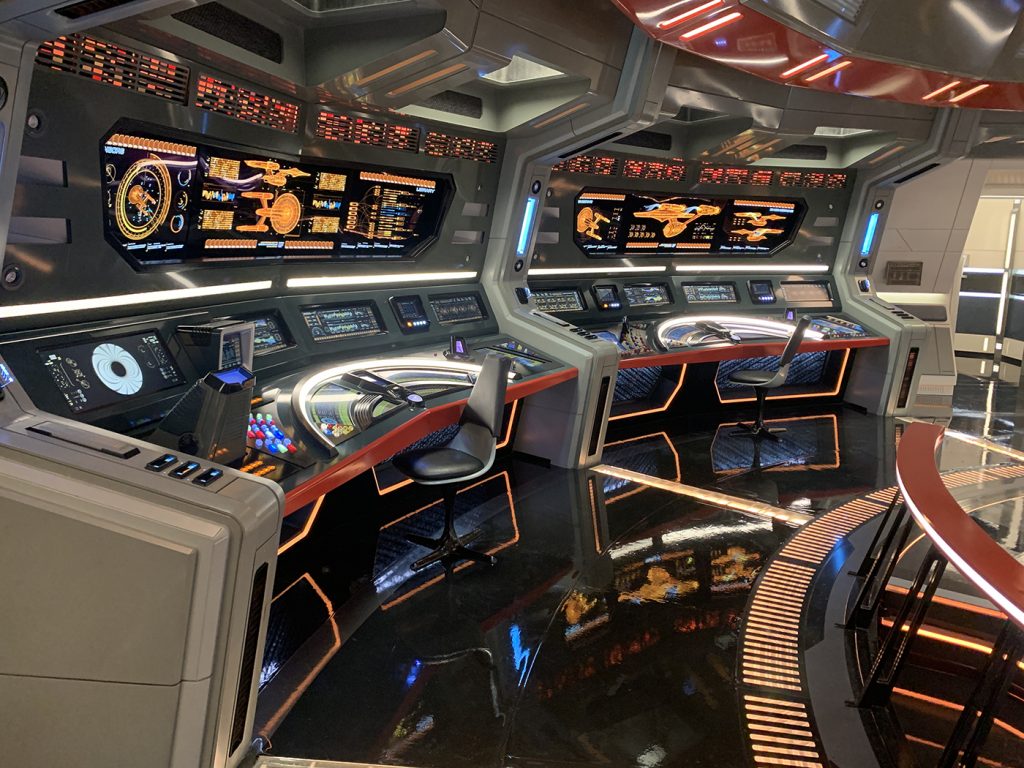The image depicts an intricate and polished control room, reminiscent of a Star Trek flight deck or a similar sci-fi environment. The room features a circular layout, adorned with complex control panels and digital displays, highlighting diagrams and statistics of a spaceship, likely the Starship Enterprise. The control panels are equipped with numerous buttons, controls, and monitors, all illuminated by predominantly orange lights, contrasted by black and gray elements. Two prominent gray chairs are positioned at the consoles, indicating where operators would sit to manage the ship's functions. The highly reflective, shiny black floor adds to the futuristic ambiance, mirroring the surrounding equipment. Additionally, there's a distinctive red railing on the right side, and the entire scene exudes a high-tech, cinematic quality, undoubtedly serving as the set of a well-known sci-fi television show.